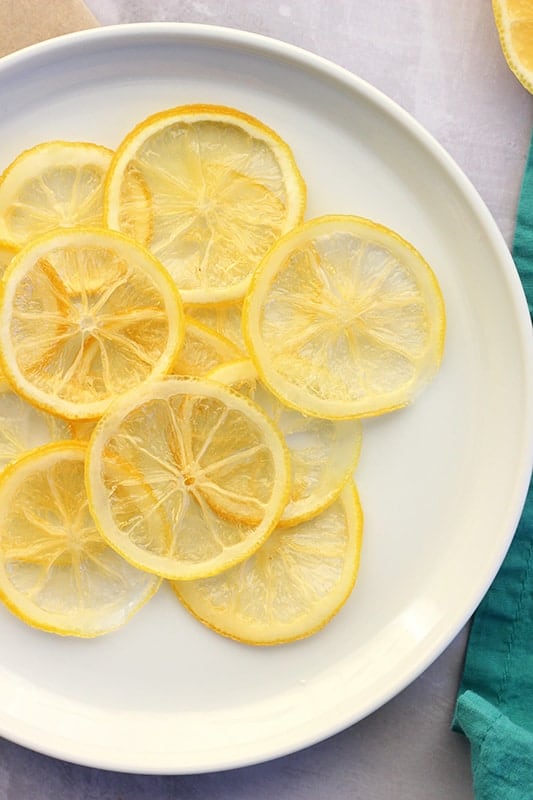The image features a white, round plate with a low rim, containing approximately a dozen very thin, see-through lemon slices. The lemons are artfully arranged, with four slices prominently displayed on top, partially overlapping each other. One slice is just left of center, another is slightly above it and to the right, a third is directly to the right and slightly below, and a fourth is below and to the left of the third slice. These are so thin they appear almost transparent, allowing several more partial slices to be visible beneath them. The plate occupies most of the image but is cut off on the left edge, with the top and bottom edges fully visible. The background is a white tablecloth, and a green napkin is seen along the right edge, extending from the bottom right corner to the top right and down to the bottom of the image. A small portion of another lemon slice is also visible in the upper right corner. The setting is bright, with clear, natural lighting, enhancing the vivid yellow of the lemons against the stark white plate and tablecloth.